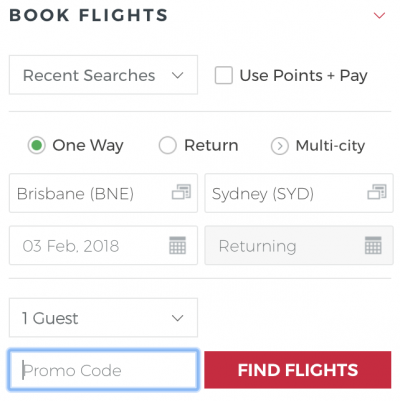The image displays a detailed view of a flight booking application interface. At the top, a bold and prominently positioned header reads "Book Flights." Directly beneath this, a tab labeled "Recent Searches" includes a drop-down arrow, likely offering quick access to previously searched routes. 

Below the Recent Searches tab, navigation options are presented horizontally: "One-Way," "Return," and "Multi-City." In this particular instance, "One-Way" is selected, highlighted in green to indicate its active status. 

The primary user interface section consists of fields for entering departure and destination locations, the departure date, and the return date, even though the immediate selection is for one-way travel. In the lower right corner of the screen, a red "Find Flights" button with white text draws attention as the next step for users to proceed with their search. Adjacent to this button is a box designated for entering a promotional code, allowing users to apply discounts to their booking.

The overall background of the application is clean and white, enhancing readability and user focus on the input fields and action buttons.